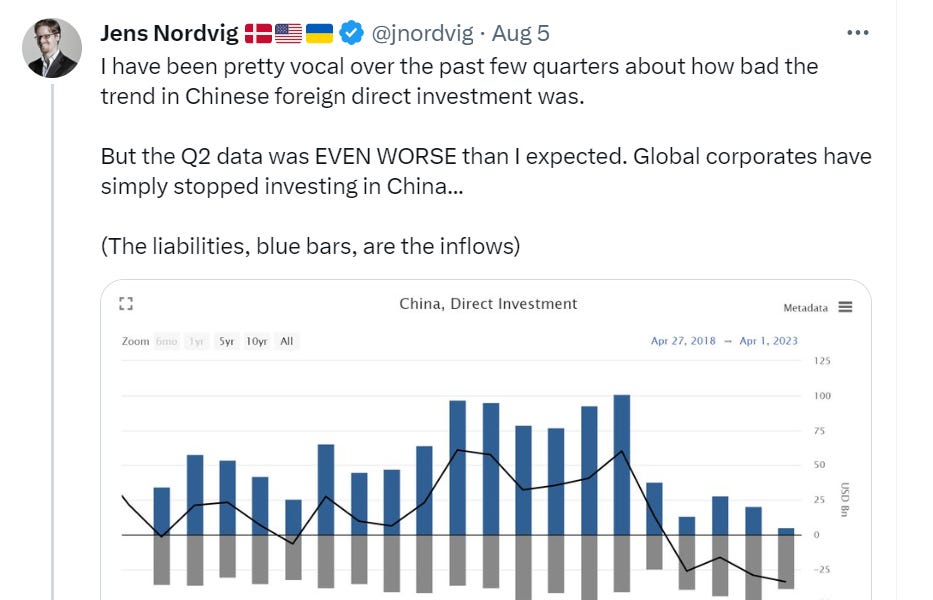**Detailed Caption:**

This social media screenshot from X.com (formerly known as Twitter) features a post by Jens Nordvig (@jnordvig), dated August 5th. The profile picture on the right side shows Nordvig turned sideways, sporting short brown hair and glasses, wearing a white dress shirt and a dark blue or black tuxedo. The background behind him is dark gray. Next to the name, Jens Nordvig, written in black, are three flags: one red with a white cross (presumably Switzerland), followed by the American and Ukrainian flags. There's also a small circle with waves and a white checkmark indicating verification status.

The post's text is in black and reads: "I've been pretty vocal over the past few quarters about how bad the trend in Chinese foreign direct investment was. But the Q2 data was even WORSE than I expected. Global corporates have simply stopped investing in China..." Below this statement is a parenthetical note: "(The liabilities, blue bars, are the inflows)." 

Accompanying the text is a bar graph where the dark blue bars extend upward and the dark gray areas decline below the graph, representing a stark contrast in data trends. A line graph intersects the blue section of the bar graph, illustrating the data trend visually.